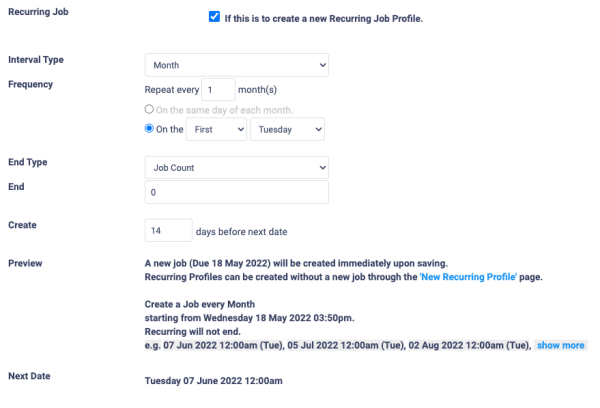This image showcases a detailed "Recurring Job" creation page. 

In the top left corner, there's a label titled "Recurring Job." Adjacent to it on the right, a blue checkbox is marked, indicating that a new recurring job profile is being created. Below, labeled sections include "Interval Type" where users can select specific months, and an option to enter the repetition frequency in months. 

Beneath this, there are two radio buttons allowing users to choose between "On the same day of each month" or "On the first [specific day]." Here, the user has selected "First Tuesday of every month." Further down, fields labeled "End Type" and "End" appear, where a job count can be specified, followed by an input for a number. 

At the bottom of this segment, there is a "Create" button, beneath which the configuration reads: "14 days before next date." 

A "Preview" button is located near text stating: "A new job due 18 May 2022, will be created immediately upon saving. Recurring profiles can be created without a new job through 'New Recurring Profile' page."

Additional instructions are provided below: "Create a job every month starting from Wednesday, 18 May 2022 at 3:50 PM. Recurring will not end." The subsequent date is listed as "Next date: Tuesday, 07 June 2020, 12 AM."